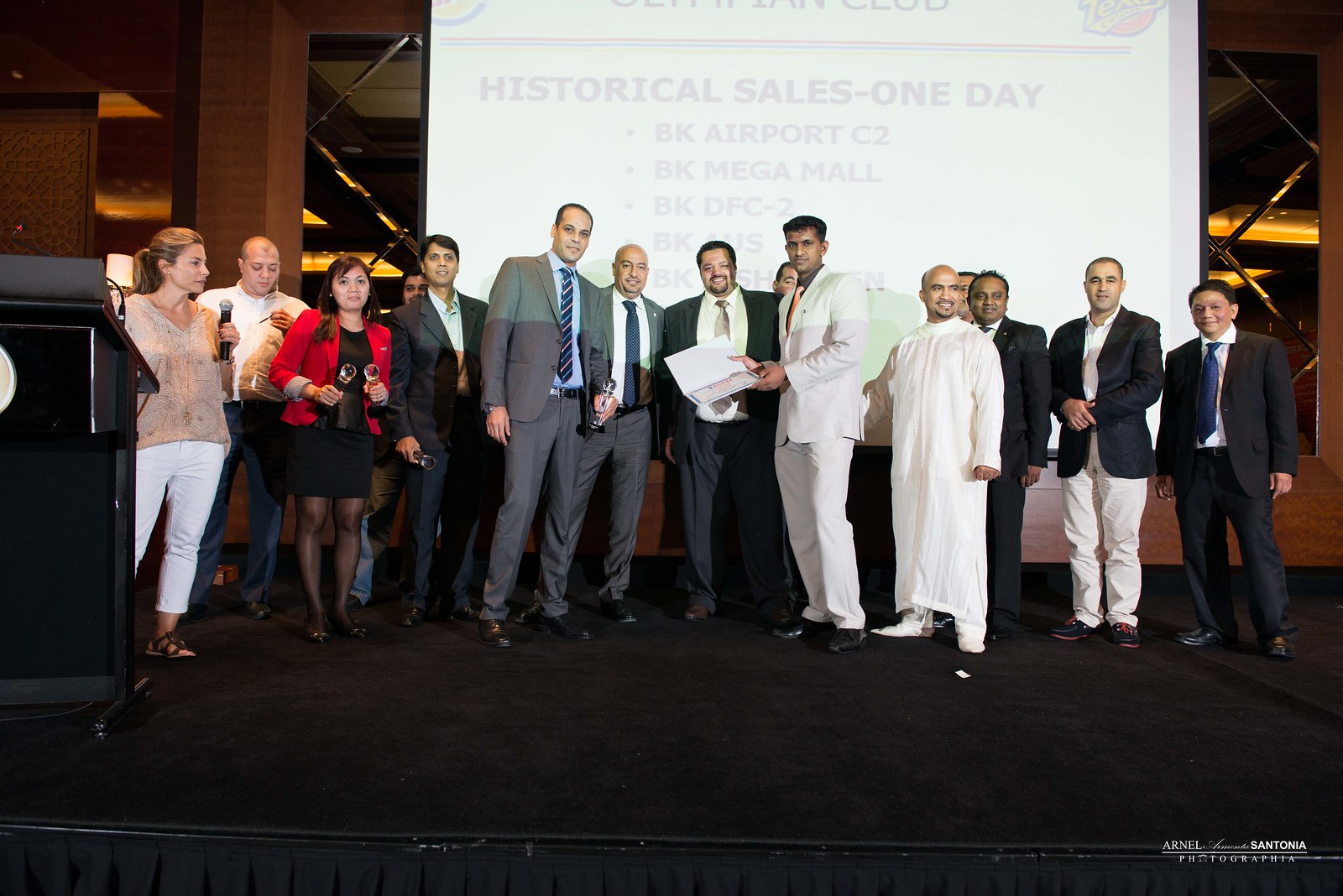The image depicts a stage at a promotional or trade event, attended by industry professionals, primarily men in suits and ties, with two women present. The backdrop features a projector screen displaying faint purple text reading "Historical Sales - One Day" along with some partially obscured text such as "BK Airport C2," "BK Mega Mall," and "BK DFC - two," indicating the event's theme. Among the individuals on stage, some hold trophies, signifying an awards presentation. Notably, on the far left, a woman in a red sweater and black dress stands behind a black podium, holding a microphone in her left hand. To her right, another woman is more casually dressed and holds two trophies. One man, distinguished by his eastern attire, wearing a long white smock and white shoes, stands out on the right side of the stage. Another tall man in the center sports a white jacket and pants, holding what looks like a certificate of recognition. The stage floor is black, and a wood-toned border surrounds a mirror or window in the background. Everyone is smiling at the camera, suggesting a celebratory atmosphere in what appears to be a large convention hall.